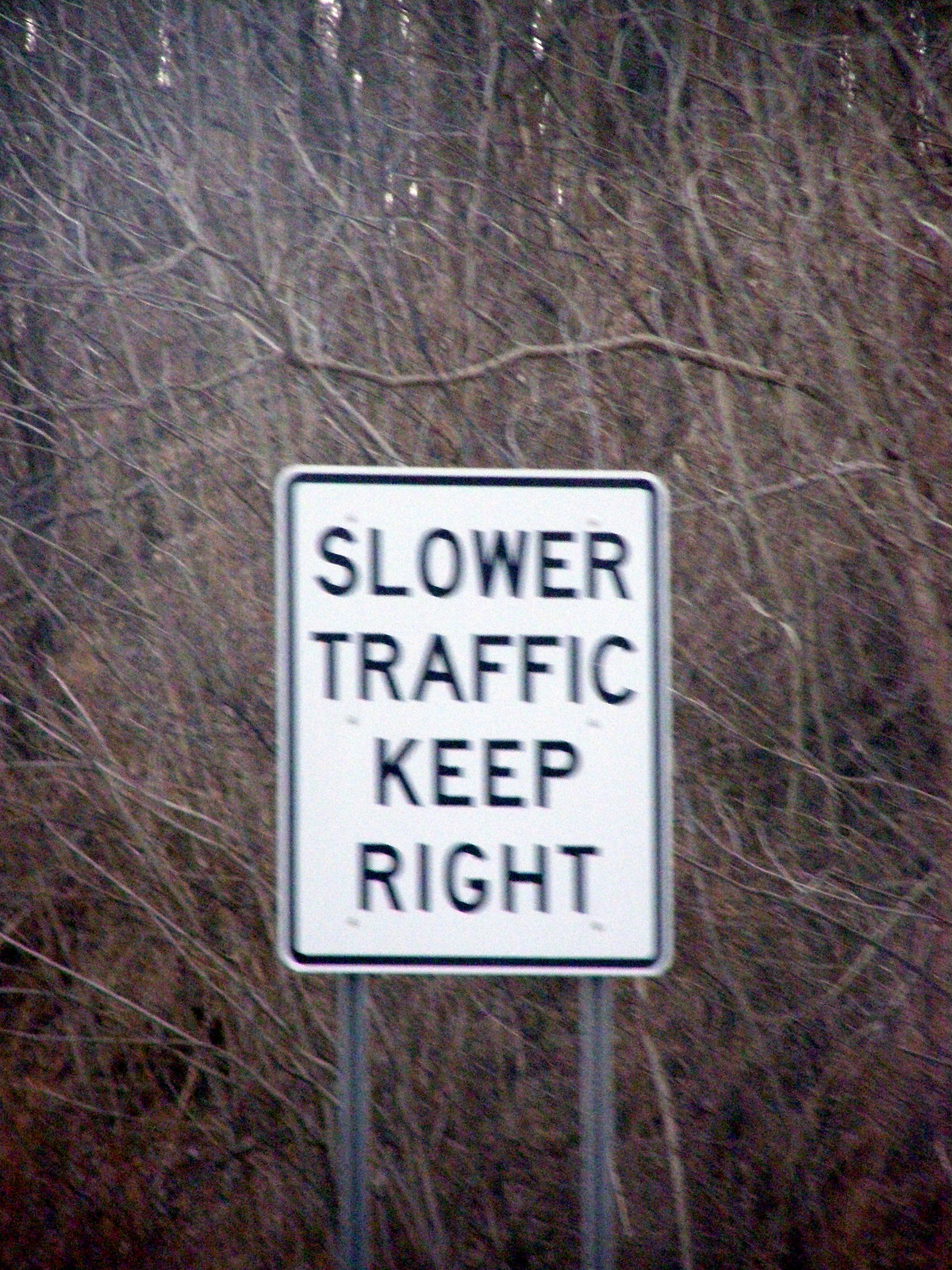This photograph captures a white rectangular traffic sign with a thin black border and bold black all-caps text that reads, "SLOWER TRAFFIC KEEP RIGHT." The sign is securely fastened with bolts to two grey metal posts that anchor it to the ground. The scene is set in a densely wooded area, where an intricate network of bare tree limbs completely obscures the sky, giving the impression of a late fall or early winter season. Most tree limbs appear to tilt towards the left, adding a unique character to the landscape. The overwhelming presence of leafless branches dominates the background, creating a nearly impenetrable thicket of twigs and limbs behind the sign. A small patch of sky peeks through the dense canopy at the very top of the image, adding a subtle touch of brightness to the otherwise rugged and natural setting.